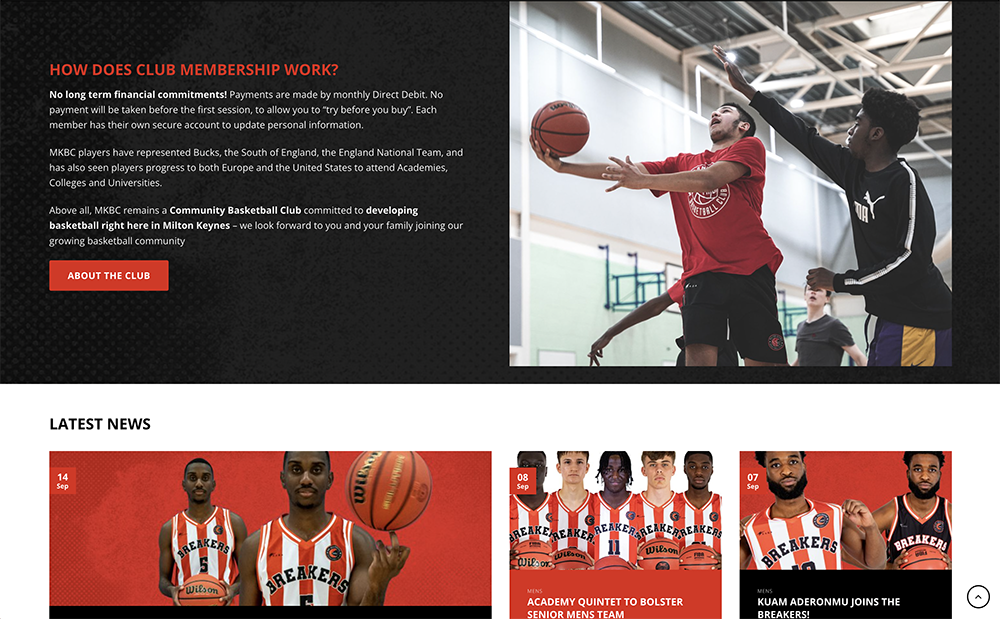The screenshot captures a section of a website, though the header graphic identifying the organization is absent. The top of the page is divided into two halves. On the right, there's an action-packed photo of two young men playing basketball. The player on the right is a dark-skinned black man wearing a long-sleeve T-shirt with a prominent white Puma logo. His opponent, likely of Hispanic descent, is dressed in a red T-shirt and dark, possibly black, shorts, and is holding the basketball while the black man attempts to steal it.

The left side of the screen has a black background featuring a red headline that asks, "How does club membership work?" Below, in white font, it states, "No long-term financial commitment." At the bottom of this section, white text emphasizes, "Above all, MKBS remains a community basketball club." Beneath this message, there's a noticeable red button labeled "About the Club," presumably leading to more detailed information about the organization.

Further down, the page displays three photos, each cropped around the elbows, of various players against brick-red backgrounds. Most of the players are black men, with a few white men among them. The team uniforms seen in these photos feature vertical red and white stripes, creating a cohesive visual theme.